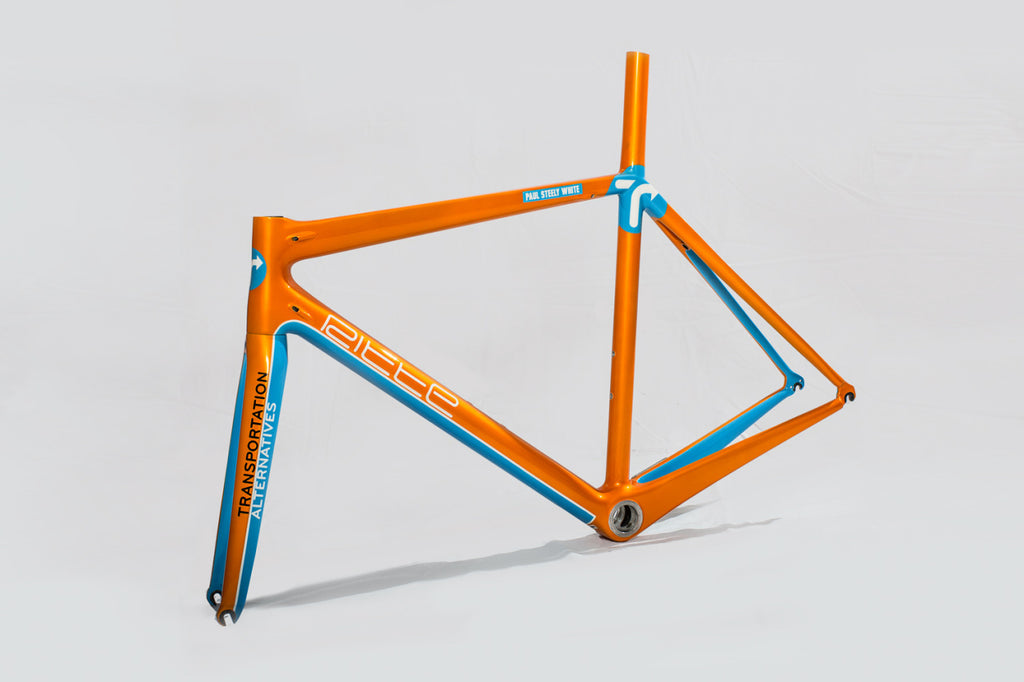This product image showcases an orange bicycle frame set against a white background, emphasizing its sleek, minimalist design devoid of any seats, handlebars, wheels, or chains. The main color of the frame is predominantly orange, accentuated with sky blue accents that trace along its edges, enhancing its visual appeal. Detailed white text reading "R-I-T-T-E" appears across the main support bar in a abstract, fluid font, adding to the frame's unique design. Additional text along the front supports spells out "Transportation Alternatives" in a combination of black and white letters. This product image highlights the bicycle frame's bold and modern aesthetic while suggesting it might offer some distinct features as an alternative to traditional bicycles.